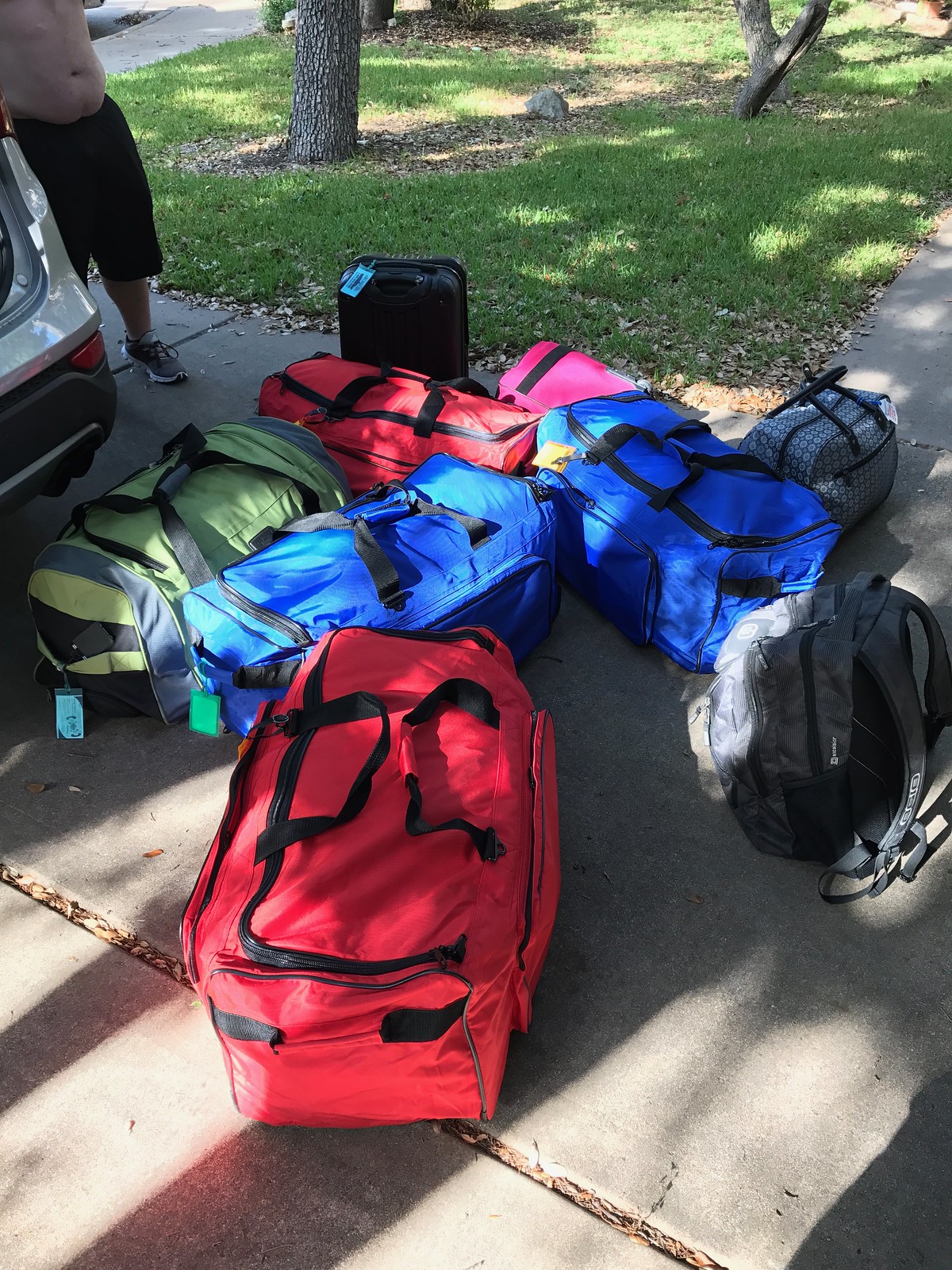This vibrant, outdoor photograph captures a busy scene centered around a multitude of bags scattered on the ground, ready to be packed into a car. Among them, we see two red duffel bags, two blue duffel bags, a light green duffel bag, a single pink duffel bag, and a black backpack. There's also a carry-on type of rolling plastic luggage. They are all strewn across the concrete driveway, which connects to the sidewalk and the lawn. In the background, a shirtless man in knee-length black shorts, possibly preparing for a trip, is partly visible. The scene is bathed in sunlight, which casts reflections on the pavement and highlights parts of the green lawn and a couple of tree trunks, their leaves casting shadows on the grass. The edge of a car is just visible, suggesting imminent travel.